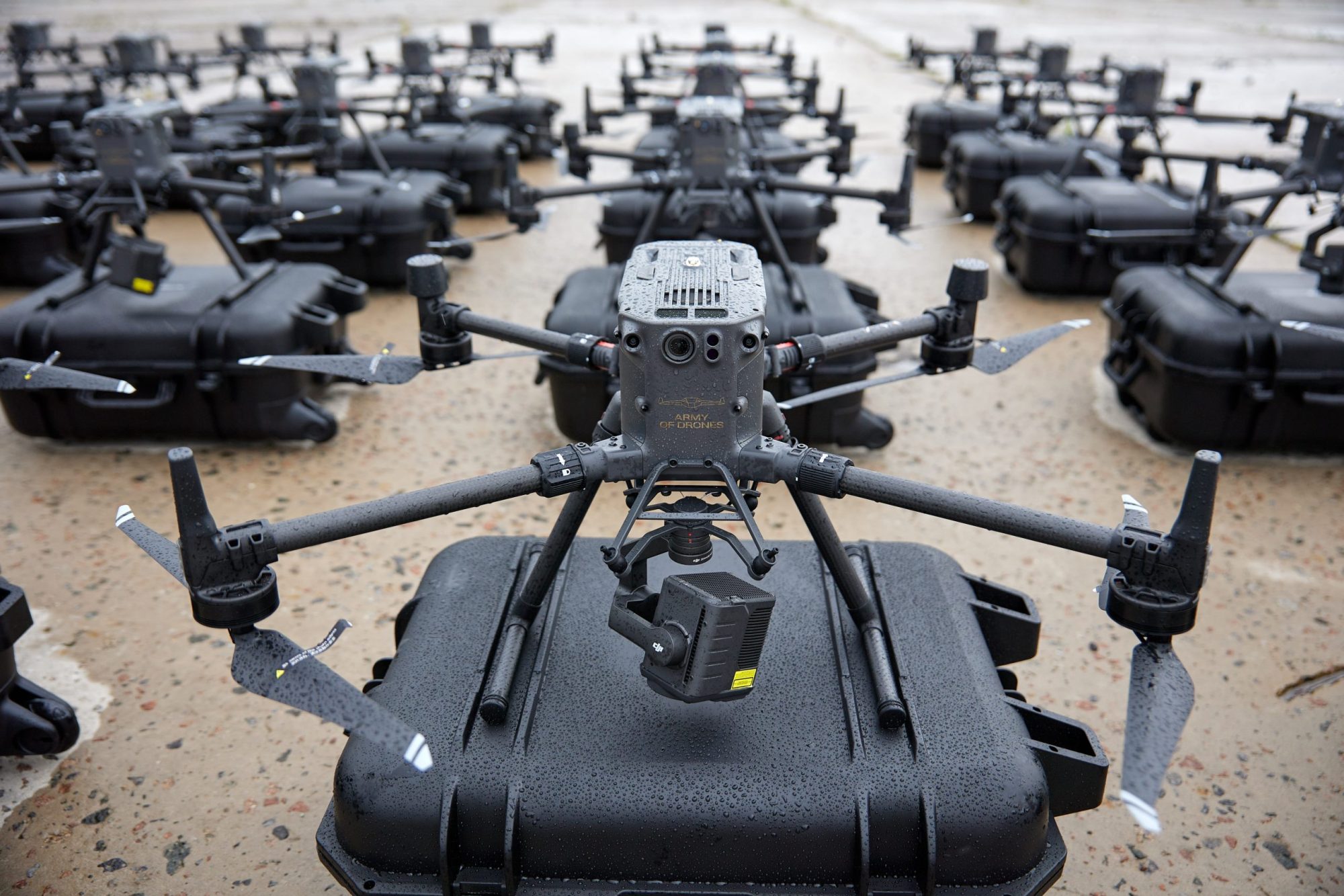The photograph captures an array of identical drones meticulously arranged in rows and columns on black, hard-plastic cases that serve as their transport containers. Each drone, characterized by its central body flanked by several lenses that lend it a bug-like appearance, features a combination of a large, central round lens, two smaller lenses to its sides, and two additional smaller round lenses extending from its face. The drones have a vertical rectangular body from which arms extend from the corners to support propellers, distinctively positioned at the bottom. Their landing gear consists of metal tubes forming a stable base. Attached to the underside of each drone is a rectangular device, possibly another camera. The drones and cases are situated on a brownish stone or concrete surface speckled with various colors, suggesting the area might have recently experienced rain. The closed black cases, equipped with handles and wheels, hint at the drones' readiness for transport or deployment. The outdoor, daytime setting underlines the preparedness and systematic arrangement of these advanced devices.